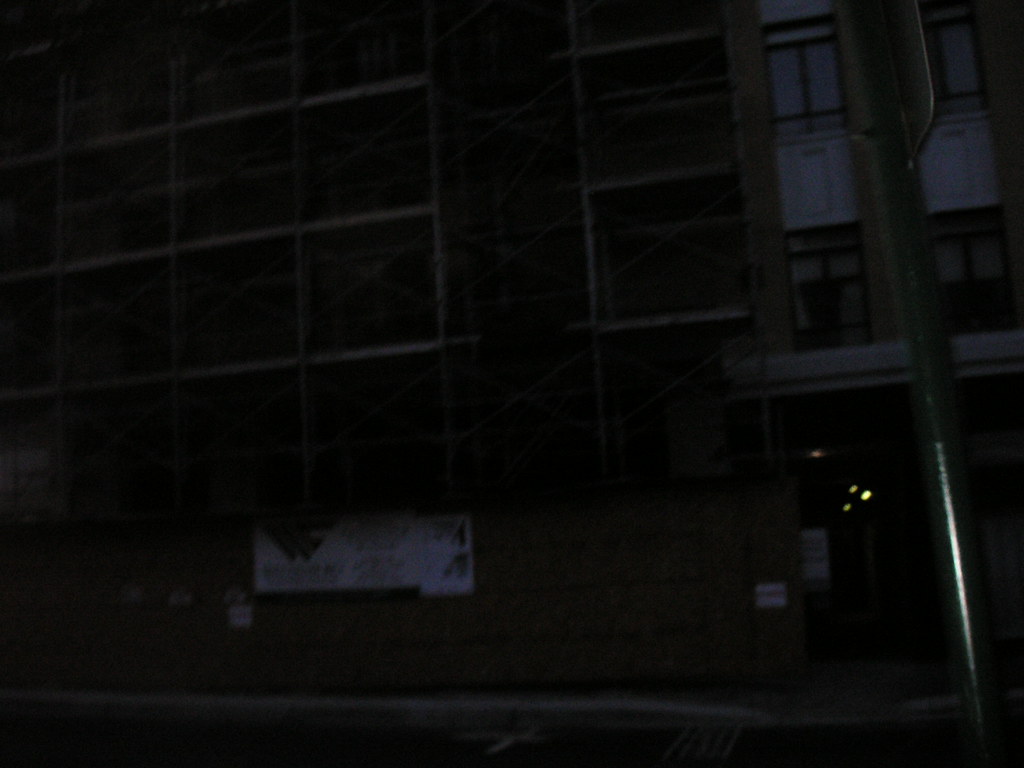This is a very dark, low-resolution image taken at nighttime, likely in motion. The scene shows a construction site with prominent scaffolding on the left side of a building. The scaffolding forms a squared grid pattern with crisscrossing X's for stabilization, starting about 10 feet up and extending beyond the top of the picture. 

In the foreground is a street intersection with a crosswalk, featuring white paint lines and asphalt paving, leading to a gray concrete sidewalk. To the right in the foreground, a green crosswalk pole stands with its sign facing left, though the front of the sign is not visible. Near the camera, a waste management bin is positioned, adding to the sense of construction work.

The building itself has closed windows and a brick wall at the lower level, ending before a doorway on the right side. This doorway is accompanied by three small lights arranged in a triangular pattern down its hallway. Above the doorway and extending upward, the scaffolding frames the structure. Reflective light from a nearby light pole adds some visibility to the otherwise dark scene. In the right background, apartment windows are faintly visible, indicating residential presence amidst the ongoing construction.